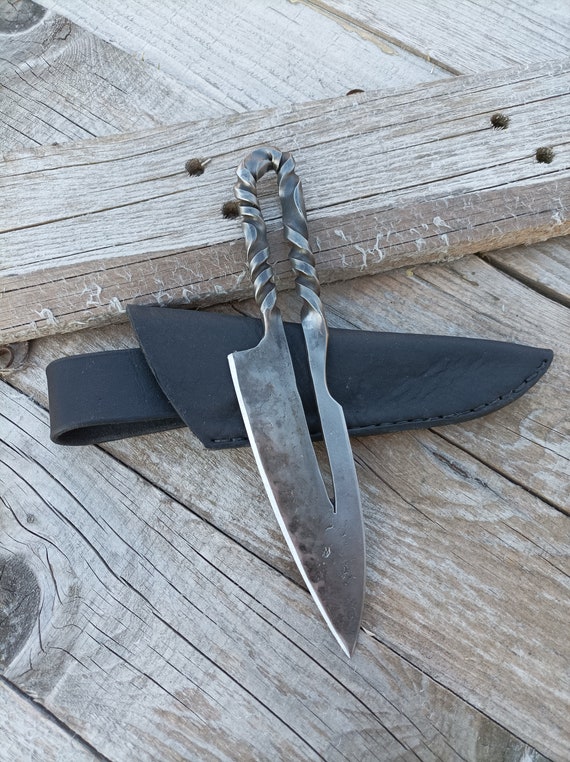The photograph showcases a horizontally aligned rectangular image divided into two major sections by a darker brown board, creating an unofficial dividing line. This board, about a centimeter thick from the viewer's perspective, runs diagonally from lower left to upper right and has a shadow and white paint splatters on its surface. Resting against this board is an antique or replica chopping knife, with the blade pointed towards the viewer, slightly to the right. The knife features a distinctive design, with a V-shaped blade that narrows into a decorative loop handle with thick spiral patterns.

Alongside the knife, there are two smaller black blades: one triangular and one rectangular, positioned beneath the main blade. These blades add to the intricate metallic composition.

In the background, there are numerous weathered wooden boards. One wider, lighter-colored board runs parallel to the darker dividing board, extending across the frame with four nails drilled in diagonally. Behind this, lighter diagonal boards extend the depth of the composition. The wood appears unvarnished and rustic, potentially resembling a picnic tabletop. Crisscrossed cloth with a light plaid pattern is faintly visible behind these boards, adding texture to the scene.

Additionally, there is a black, leather knife sheath with a strap, suggesting the knife could be attached to a belt. This sheath and the knife rest together on the various wooden boards, creating a complex and detailed visual arrangement that combines metallic elements and textured wood.